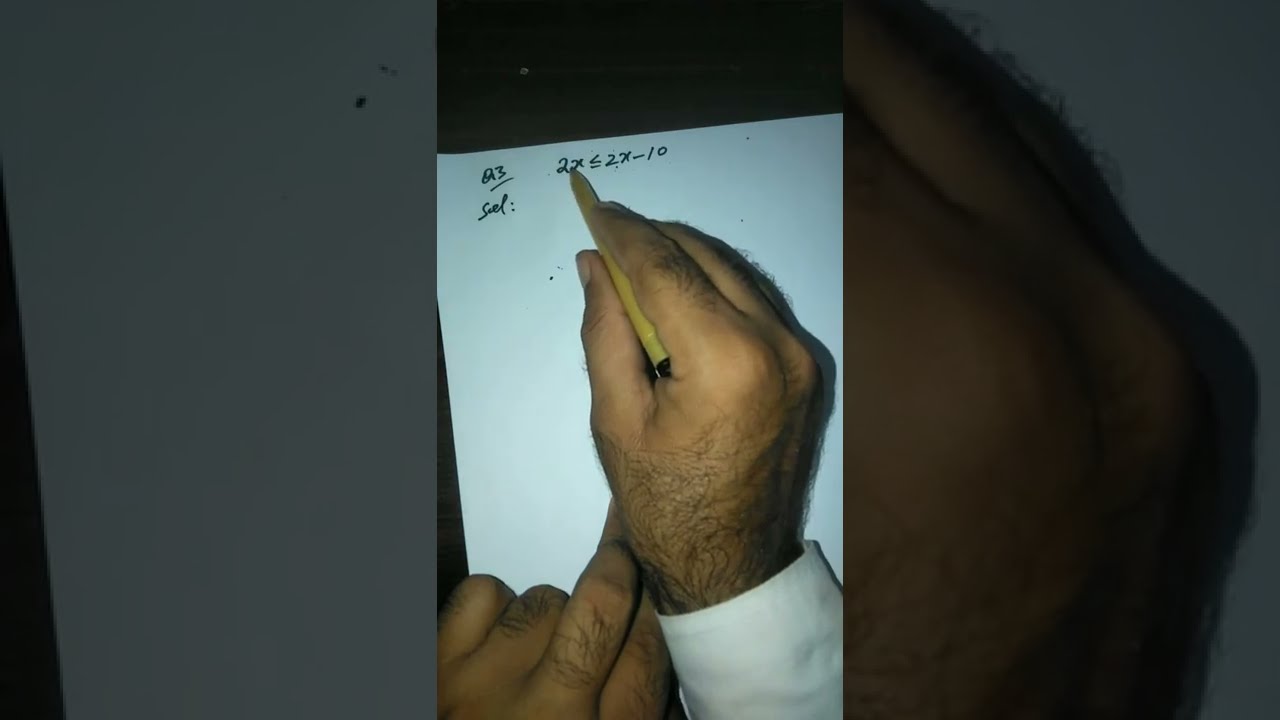This is a horizontally oriented photograph characterized by a somewhat darker tone. Central within the image, a man's hands—remarkably hairy—are prominently featured against a blank piece of white paper. Occupying the middle section, his right hand holds a short brown pencil or pen, used to write mathematical equations. The visible script includes "2x ≤ 2x - 10," as well as possible partial equations like "23" or "Q3" and "solve:" though portions are indistinct. His hands emerge from the bottom of the image, adorned in a long-sleeve white dress shirt. To the left and right of this central focus are close-up segments: the left depicts a blank part of the paper, while the right provides a detailed view of his right hand and knuckles. Additionally, this primary scene is superimposed upon an enlarged and somewhat grayscale background of the same image, contributing a layered, collage-like effect. The photograph is slightly cropped at his wrists, adding to the intimate, focused atmosphere of the composition.